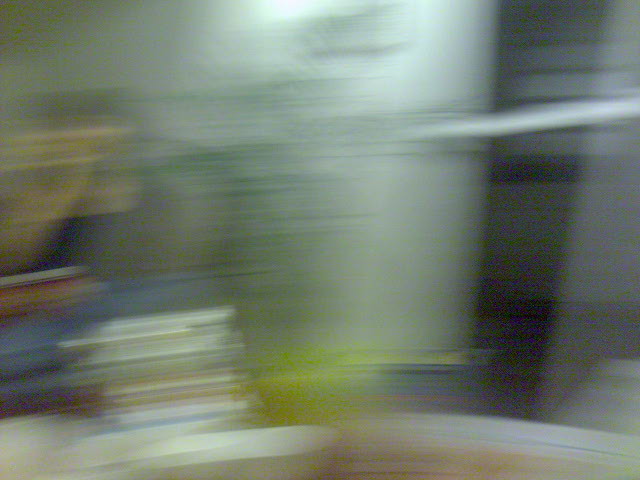The photograph is exceptionally blurry, rendering it a chaotic blend of colors with a significant motion blur effect. Dominant hues include white, green, blue, yellow, black, silver, and tan, swirling and streaked across the image as though captured with a moving camera. In the background stands a white wall accented by a green plant stretching upwards, creating staggered green lines amidst the blur. A cluster of objects that could be books sits on what appears to be a tabletop, adding to the cluttered scene. A tall black shape, possibly a doorway to a darker room, is visible in one corner. Also noticeable are distinct color streaks: a blue streak mingles with yellow and white streaks, forming a layered, dynamic color pattern. Amidst these blobs and streaks, vague shapes hint at the outline of a person or an animal, adding to the overall enigmatic and abstract quality of the image.